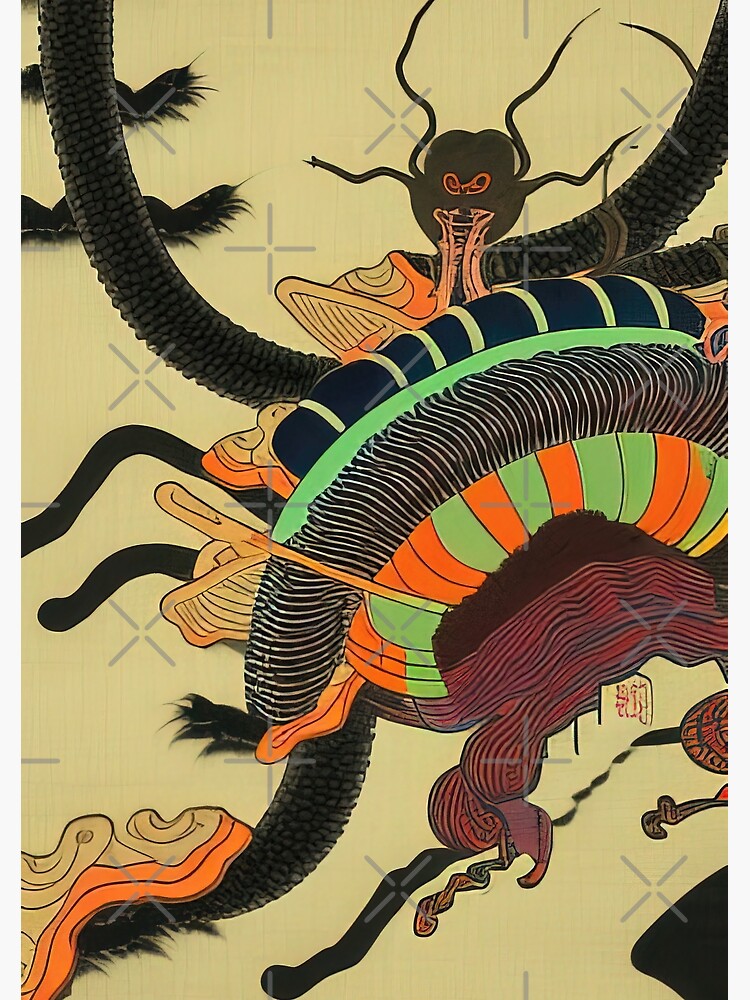This detailed painting appears to merge various cultural and abstract elements to create a visually complex scene. At the center, a prominent brown mask with four curved, wavy spikes extends from the sides, possibly signifying a form of spiritual or cultural symbolism. The mask, with red eyes and incomplete, artifact-like features, suggests an AI-generated feel, adding an eerie, surreal quality to the artwork.

Beneath this mask, an array of vibrant colors and shapes are present, dominated by a large, circular green and orange element that could symbolize clothing or a dress-like structure enveloping the scene. Intertwined among these colors is a striking black snake-like creature, characterized by black and white stripes reminiscent of dense zebra patterns. This creature appears to be twirling off to the left and swirling around the top of the painting, adding a sense of motion and fluidity.

The background of the piece maintains a faded white hue, highlighting other intricate details such as gray X’s scattered throughout the image. All these elements combine to create a richly textured, abstract composition that evokes interpretations from African and Japanese traditional styles, making it a unique fusion that captures the viewer's imagination.